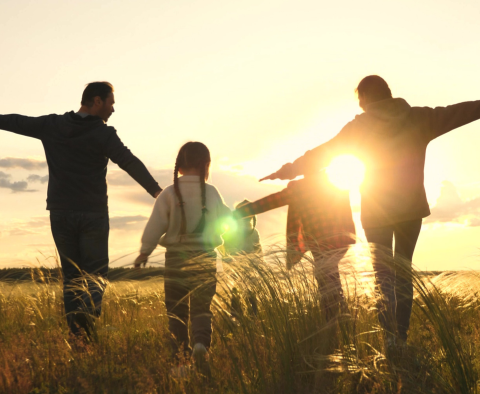In this captivating photograph, a family of five is captured walking through a field of tall, ember-colored grass during the golden hour of sunset. The family, consisting of a father, mother, and three children, is walking away from the camera. The father stands to the left, wearing dark clothing, while the mother is on the right in a grayish hoodie. Between them are their three children: a little girl with pigtails on the left, the smallest child in the middle holding a container, and another child on the right. The children and the parents, except for the daughter with pigtails, have their arms outstretched, mimicking the pose of airplanes in flight, adding a sense of playful movement. The sun, positioned near the horizon, peeks through the gaps between the family members, casting a warm, yellow and orange glow over the scene. The vibrant sunset is adorned with purple-tinted clouds, creating a magical and brightly lit yet simultaneously shadowy atmosphere. The angle of the shot, taken from nearly knee-level, emphasizes the children's perspective against the towering adults and the vast expanse of tall grass.